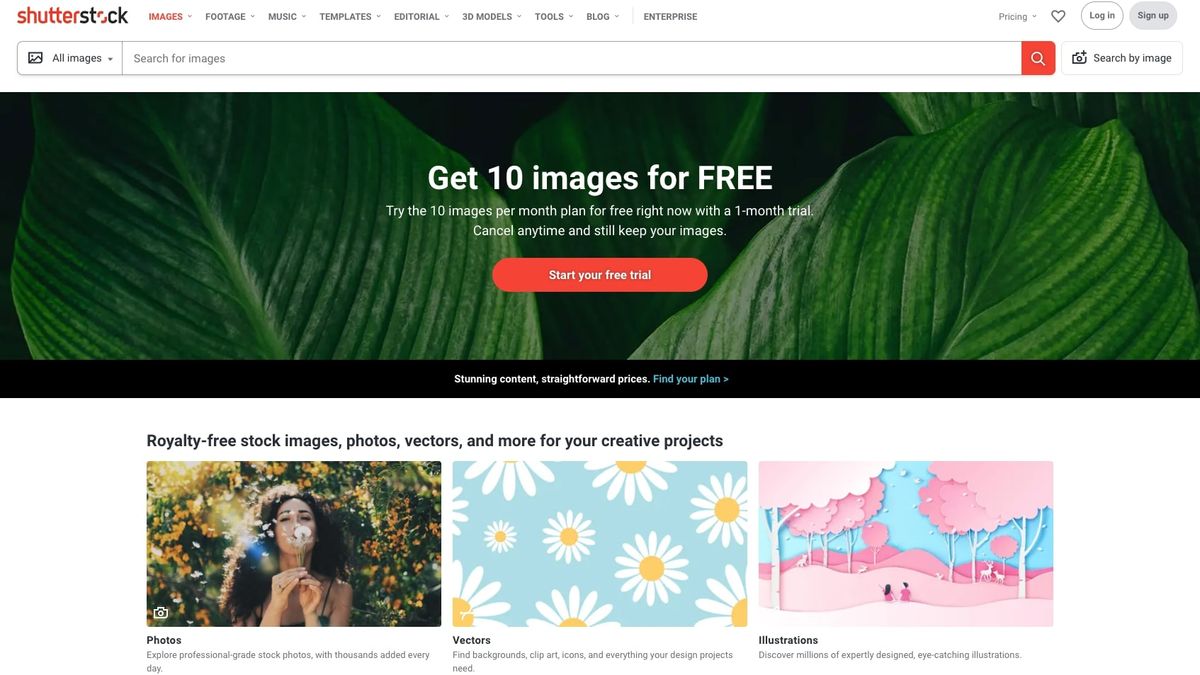This image is a detailed screenshot of the Shutterstock website, showcasing its desktop interface, characterized by a broad, high-resolution display. At the very top of the screen, the Shutterstock logo is prominently featured, accompanied by navigation links to various sections such as "Images," "Footage," "Music," "Templates," "Editorial," "3D Models," "Tools," "Blog," and "Enterprise."

Directly beneath these navigation options, a lengthy search bar spans the width of the screen, currently set to search across "All Images." The search bar includes a drop-down menu to narrow down categories and a button labeled "Search by Image," which allows users to upload an image to find visually similar content.

The central focus of the screenshot is a large promotional banner advertising a free trial offer. The banner reads: "Get 10 images for free" and continues with an enticing offer: "Try the 10 images per month plan for free right now with a one month trial. Cancel any time and still keep your images." Below this text, a prominent "Start your free trial" button invites users to take advantage of the offer.

Directly beneath this promotional banner, thumbnails of various types of visual content are displayed, including photos, vectors, and illustrations, demonstrating the range and diversity of available media on the Shutterstock platform.